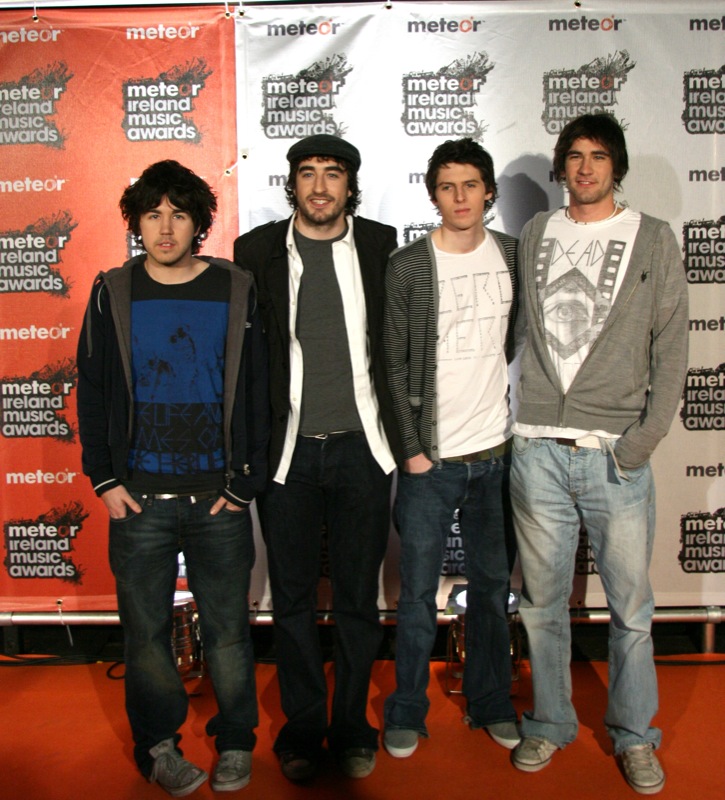In this vibrant, full-color photograph taken likely indoors under bright lights, as indicated by the shadows, four young men with dark hair and casual attire stand closely together, perhaps with their arms draped around one another, suggesting camaraderie or group unity. All appear to be in their mid-twenties and potentially part of an Irish band, given the event backdrop emblazoned with "Meteor Ireland Music Awards" repeatedly in orange and white graphics. Their outfits consist predominantly of blue jeans, sneakers, and layered tops including t-shirts, hoodies, or sweaters. Specific details include one man wearing a black t-shirt with blue logoing and a sweater, another in black pants with a layered look of a gray undershirt, a white shirt, a suit jacket, and a cap with a supple beard. The third individual dons a white shirt with a black striped overshirt and jeans while the last man sports light jeans, gym shoes, a gray sweater, and a white shirt. They stand on an orange carpet or flooring in front of this promotional billboard, adding to the sense of a formal yet relaxed atmosphere at a notable music event.